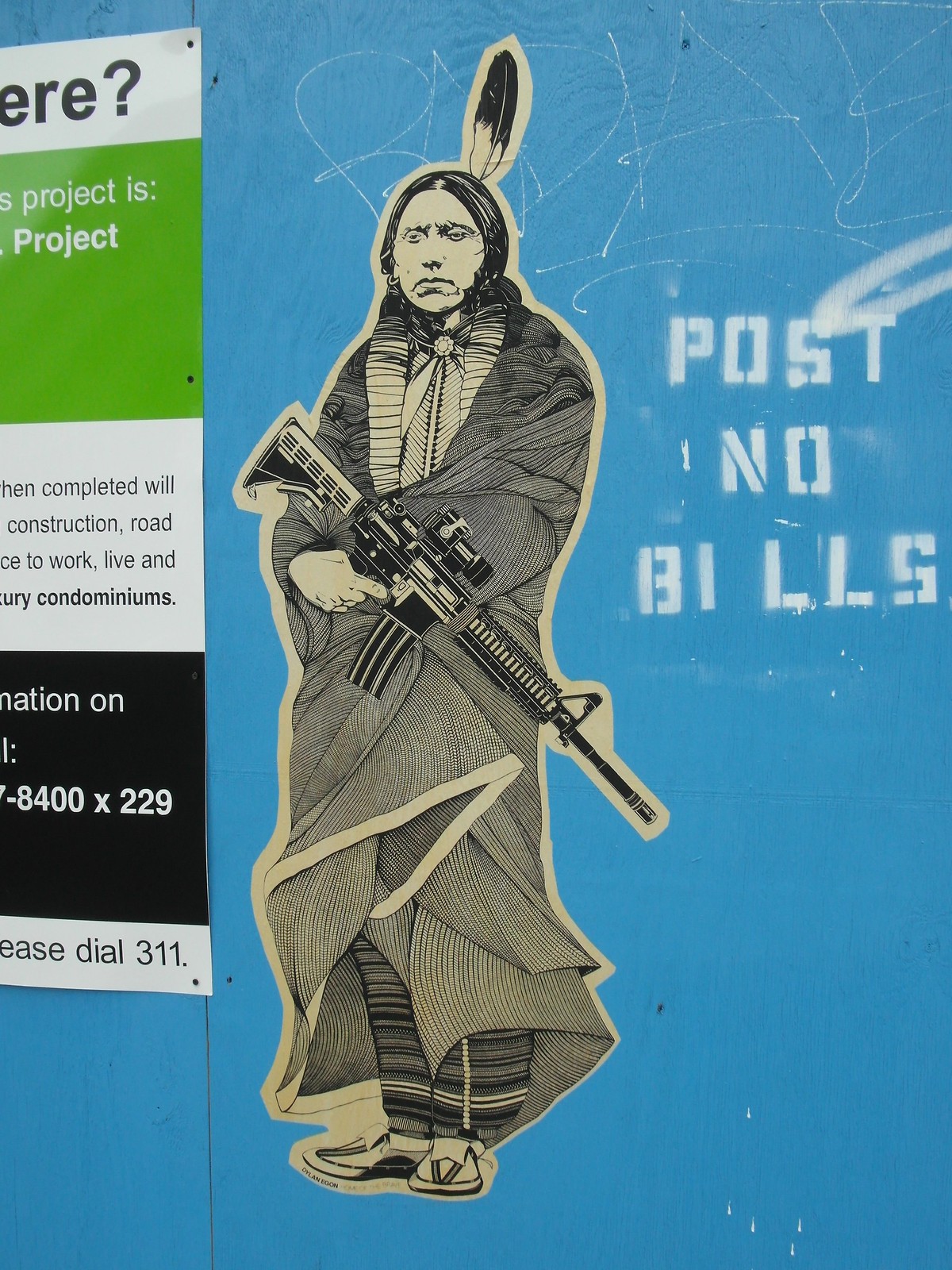The image depicts a construction site barrier made of blue plywood, commonly used to enclose building areas. On the right-hand side of the barrier, there is a stenciled message in white that reads "POST NO BILLS." Adjacent to this, there is a large, detailed sticker artwork of a Native American man. The man, with stoic expression, wears a traditional black and white ensemble that includes a long robe and striped pants. He has a black and white feather in his hair and moccasin-like sandals on his feet and is holding an M4A1 assault rifle. To the left of this figure, there is a partially visible sign with green, white, and black text, likely related to the construction project, including a fragmentary phone number "8400 extension 229" and an instruction to "please dial 311."